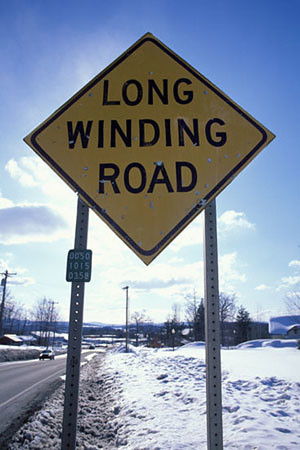The image features a diamond-shaped yellow road sign with a black border. The sign bears the bold, capitalized black text "A LONG WINDING ROAD," with each word stacked vertically. The sign is supported by two metal poles, and to the left of the leftmost pole, there is a small green sign displaying a numerical sequence: "005010150158." The background reveals a wintry outdoor scene, with visible snow patches on the right side and a road on the left, along which a small car is approaching from a distance. The landscape includes barren trees alongside fuller, evergreen trees that resemble Christmas trees. Further back, majestic mountains are visible under a blue sky adorned with scattered white clouds.